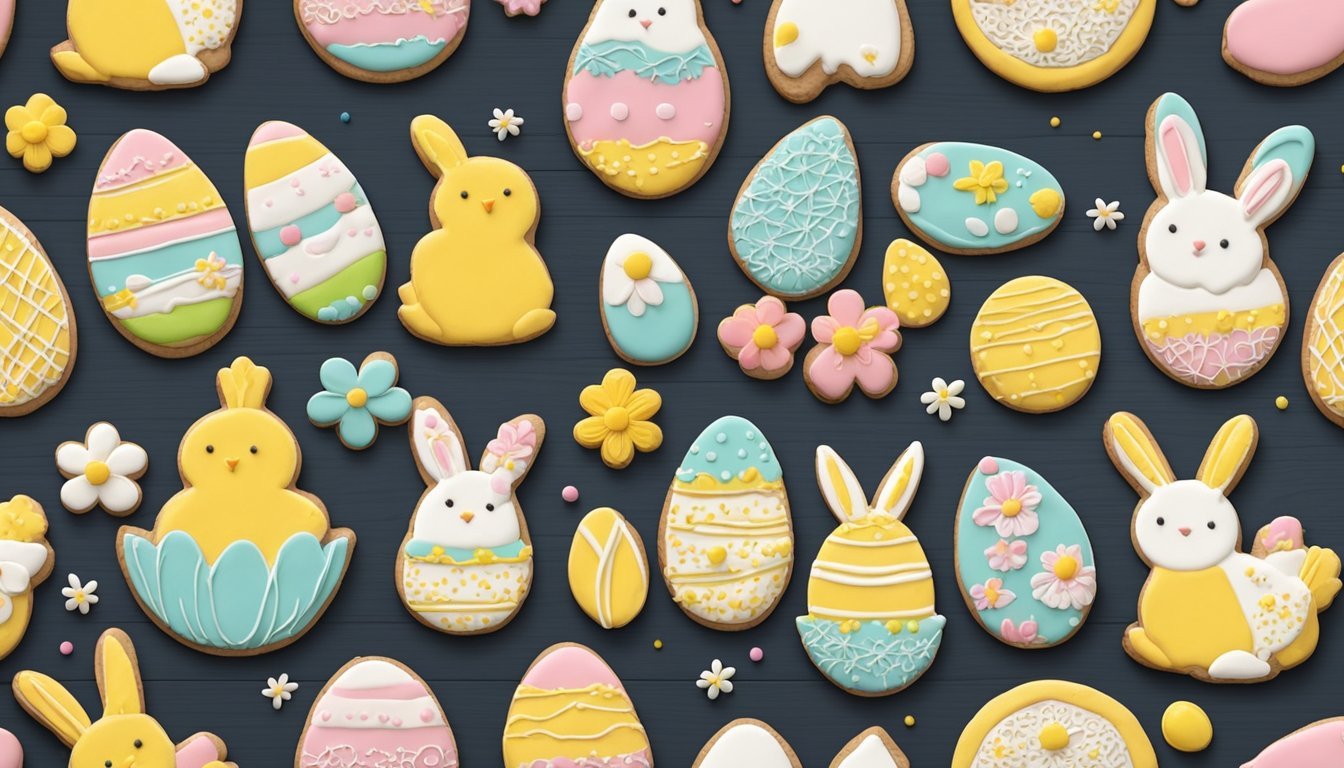This detailed, professionally staged, full-color close-up photograph showcases a delightful array of Easter-themed cookies set against a dark blue, almost black, background. The cookies, which look like shortbread, are vibrantly decorated in pastel colors—yellows, pinks, blues, greens, and whites. Various shapes can be seen, including oval cookies designed as Easter eggs with horizontal stripe patterns, as well as cookies shaped like bunnies, some painted entirely in yellow or with yellow bodies and white faces. There are also chick-shaped cookies, some appearing to pop out of scalloped edges. Interspersed among the cookies are small flowers, some looking like they are made of icing, while others resemble real white flowers with yellow centers. This visually appealing assortment gives off a cheerful springtime vibe, with each element meticulously placed to enhance the festive Easter theme.